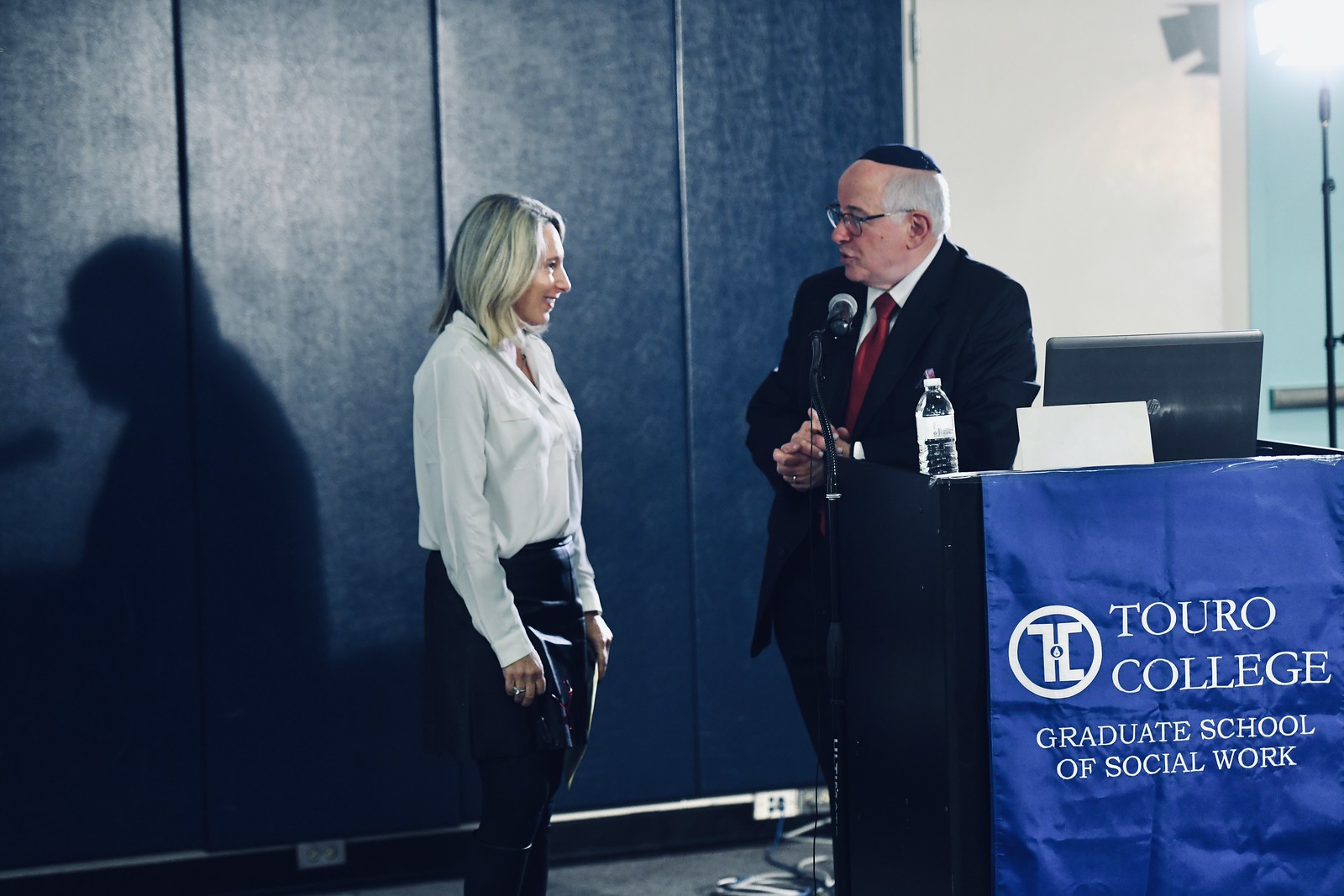The image depicts a color photograph in landscape orientation, featuring a small stage with a man and a woman engaged in conversation. The background consists of blue vertical paneling on the left and transitions to a white wall on the right. The man, positioned behind a podium adorned with a blue banner reading "Touro College, Graduate School of Social Work," is attired in a dark suit, white shirt, and deep red tie. He has short gray hair, wears glasses, and a yarmulke. His hands are folded in front of him as he speaks into a microphone. On the podium, there is an open laptop, some papers, and a bottle of water. The woman he is addressing stands facing him; she is around 50 years old, with shoulder-length silvery blonde hair, wearing a white blouse and blue pants. The setting, detailed with a spotlight in the upper right corner, exudes a formal, academic atmosphere.